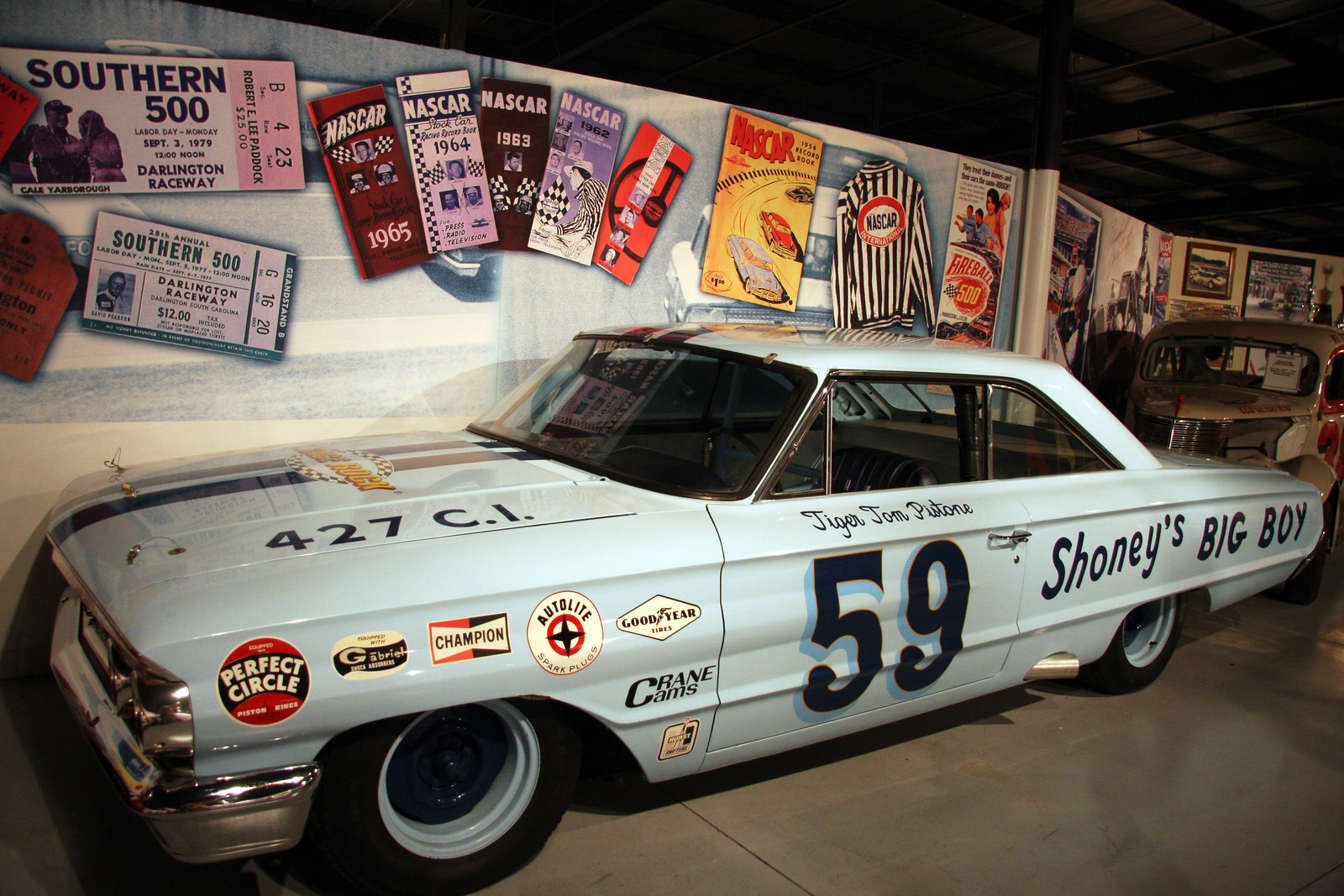This image features a classic Ford Galaxy NASCAR race car, primarily off-white with baby blue hues. The car, notable for its number 59 on the door, belonged to the famous driver "Tiger" Tom Pistone. The number 59 is displayed in blue, with the passenger side of the hood adorned by a dark blue stripe running its length. A striking orange circle with white lettering on the front fender reads "Perfect Circle." Additional decals from former sponsors such as Shoney's Big Boy, Champion, Auto Light, and Goodyear decorate the car.

The car is showcased in a showroom setting, positioned broadside with the front facing left. Behind it, a poster board highlights historical NASCAR events and memorabilia. Among these are race tickets from the Southern 500 at Darlington Raceway, varying in color and price, with notable years like 1962, 63, 64, and 65. An orange ticket and a pink $25 ticket are also visible. The background includes a NASCAR poster, a Fireball 500 poster, and a referee outfit. This detailed setup provides a nostalgic tribute to the rich legacy of NASCAR racing in the 1960s.